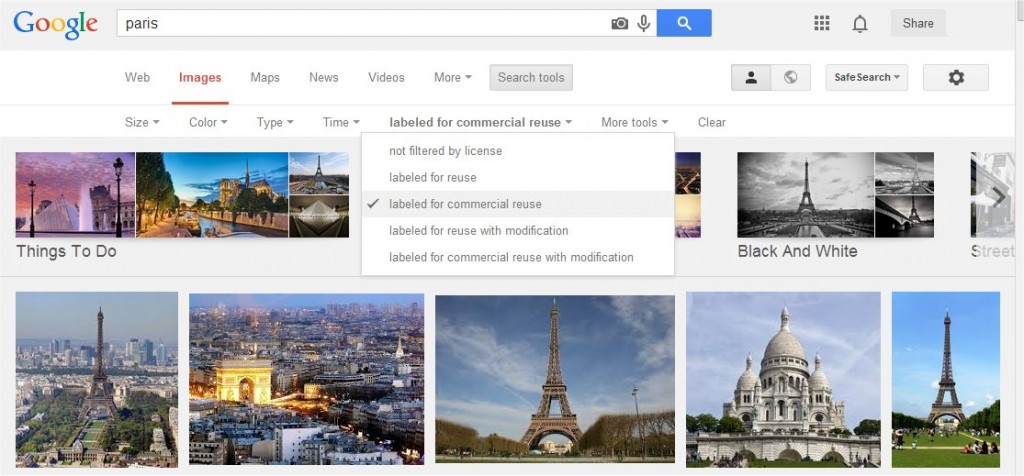This screenshot captures a Google search results page. At the top left, within a gray header, is the iconic Google logo featuring its characteristic blue, red, yellow, and green colors. Adjacent to the logo is a prominent white search bar containing the query "Paris," flanked by a small microphone icon and an image icon. To the right of the search bar are notifications and share icons. 

Below this header is the navigation bar consisting of several categories: Web, Images, Maps, News, Videos, and More, along with a gray "Search tools" option. SafeSearch is enabled, as indicated by a clickable setting positioned on the far right. Users can filter results using various criteria such as size, color, type, time, and licensing options like "labeled for commercial reuse". There is also a dropdown menu to refine search results by license type, including options like "not filtered by license," "labeled for reuse," "labeled for reuse with modification," and "labeled for commercial reuse with modification."

Further down, there are suggested filters including "things to do" and "black and white." Displayed prominently are several images, most showcasing the Eiffel Tower. One particular image stands out, featuring the Arc de Triomphe illuminated at dusk.